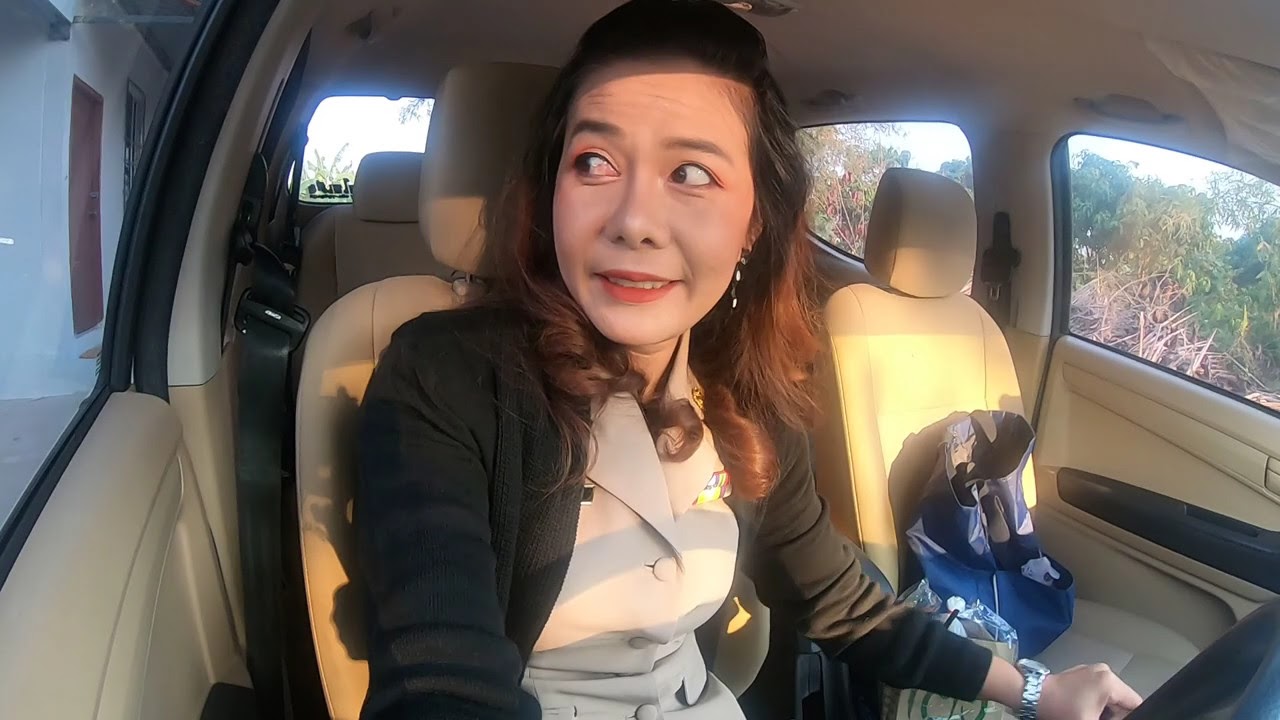This image features a woman of probable Asian descent seated in the driver's seat of a British-style car, which places her on the right side of the photograph. She has pale skin and long, brown hair, and is seen gazing out the window to her left with a subtle smile on her face. She wears a green button-down shirt layered beneath a black cardigan, and a silver watch on her left wrist. The car's interior is a yellowish beige or tannish color. To her right, on the passenger seat, lies a blue purse with a white design. The scenery outside the vehicle reveals trees and plants, and a white wall of a building on the left side of the image, along with a blue sky and additional greenery visible through the windows.